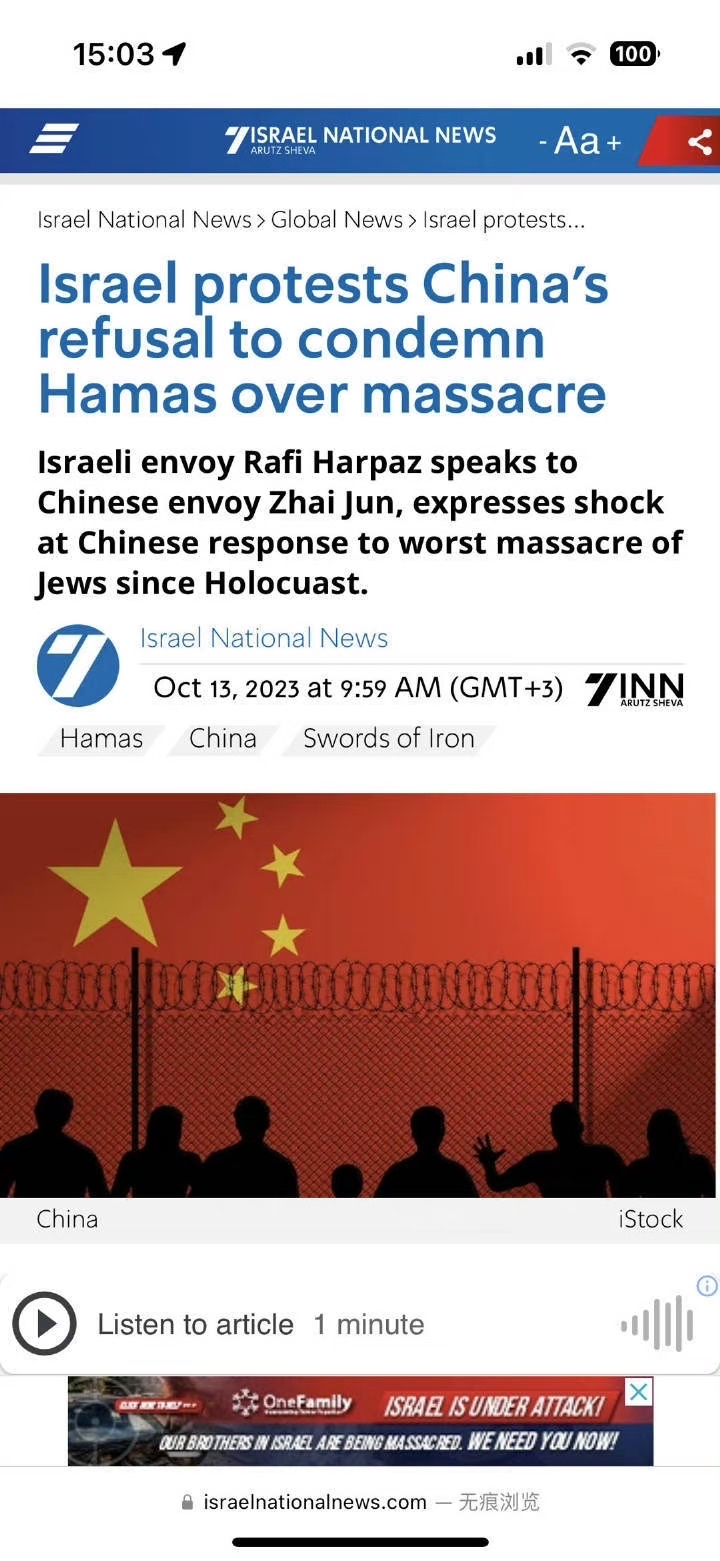**Detailed Caption for the Screenshot from the News Article:**

The screenshot captures a news article with a timestamp of 15:03 at the top, accompanied by icons for high signal, battery, and WiFi, along with a value of $4.00. The article is from "Indiegogo National News," indicated by a blue banner at the top center, which also features a share button on the far right.

Below the banner is a category section listing "Israel," "National News," "Global News," and "Israel Protests." The article's headline, written in blue, reads: "Israel Protests China's Refusal to Condemn Hamas Over Massacres." The subheadline adds more context: "Israeli envoy Rafi Hafez speaks to Chinese envoy Zha Jun, expresses shock at China's response to the worst massacre of Jews since the Holocaust."

Further down, a numeric indicator "7" suggests the TV station or channel. Next to it, "Israel National News" is displayed, followed by the date and time: "October 13th, 2023 at 9:59 AM from 7 AM." A short menu lists topics such as "Hamas," "China," and "Iran."

The central image is prominently red with a yellow star, encircled by four smaller stars, hinting at the Chinese flag. This background evokes an orange, sunset-like feel. The image also depicts a tall fence with silhouettes of various figures—men, women, and children—blacked out, possibly symbolizing a protest or a somber scene.

At the bottom, icons for listening to the article are present, accompanied by a banner with the message: "One Family Israel is Under Attack. Our brothers in Israel are being massacred. We need you now." The link to "Israelnationalnews.com" and some text in Mandarin follow the message, indicating an international audience or source.